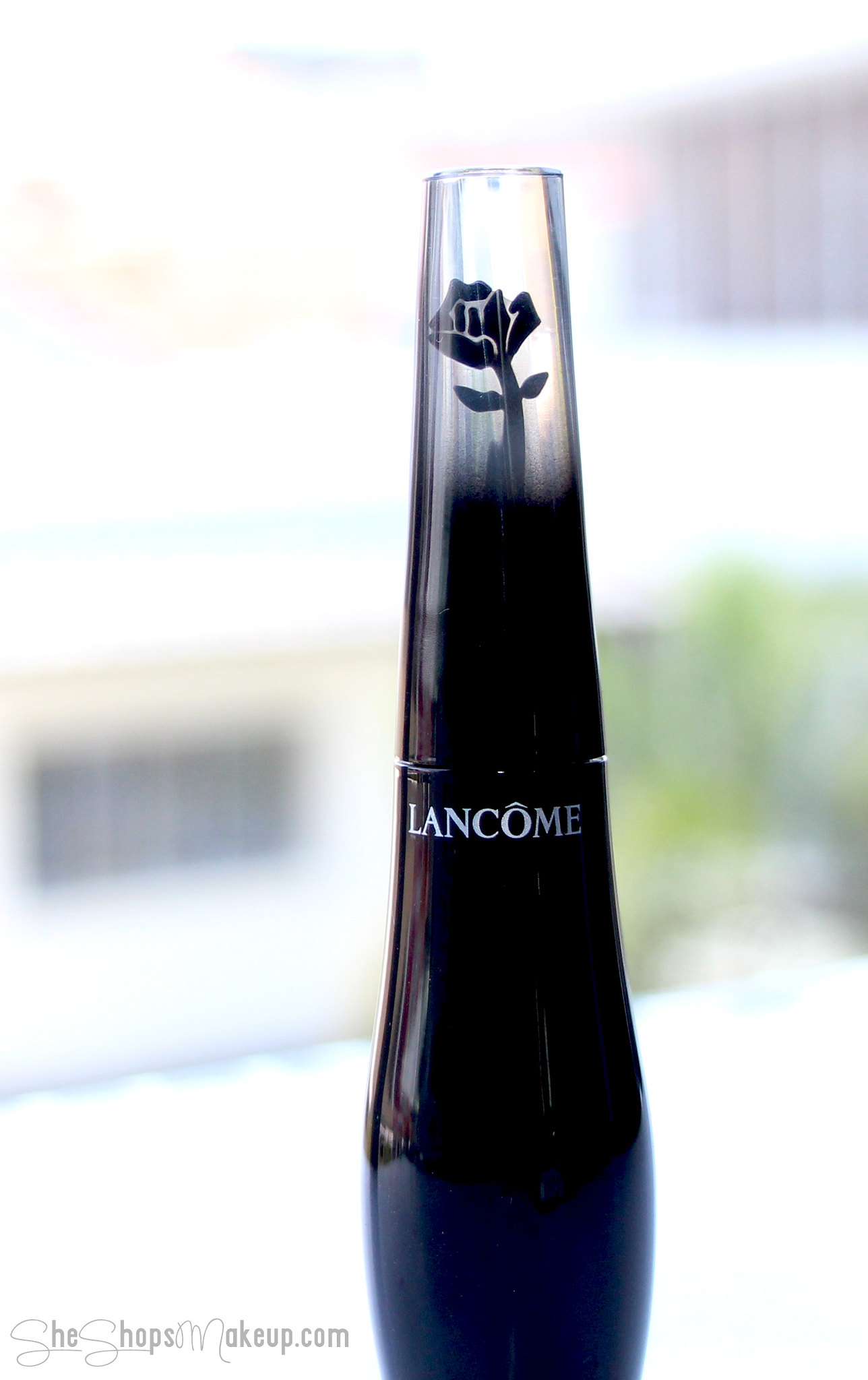The image is a close-up advertisement for a beauty product, specifically a Lancome bottle, prominently centered in the composition. The bottle is black at the base, widening slightly before tapering towards the top where it transitions into a clear, glass-like section. At the separation point, just below the cap, the brand name "Lancome" is clearly displayed. The bottle's design features a striking black rose silhouette that extends from the base upwards into the transparent section. The cap at the top is silver, accentuating the elegant and slender form of the bottle. The background is highly diffused with bright light, possibly sunlight, rendering it blurry and indistinct, though vague shapes suggest the presence of a window or building and some greenery to the right. The bottle appears to be placed on a plain white surface, creating a subtle shadow. At the bottom left corner of the advertisement, the text "SheShopsMakeup.com" is faintly visible, inviting viewers to visit the website for more details.